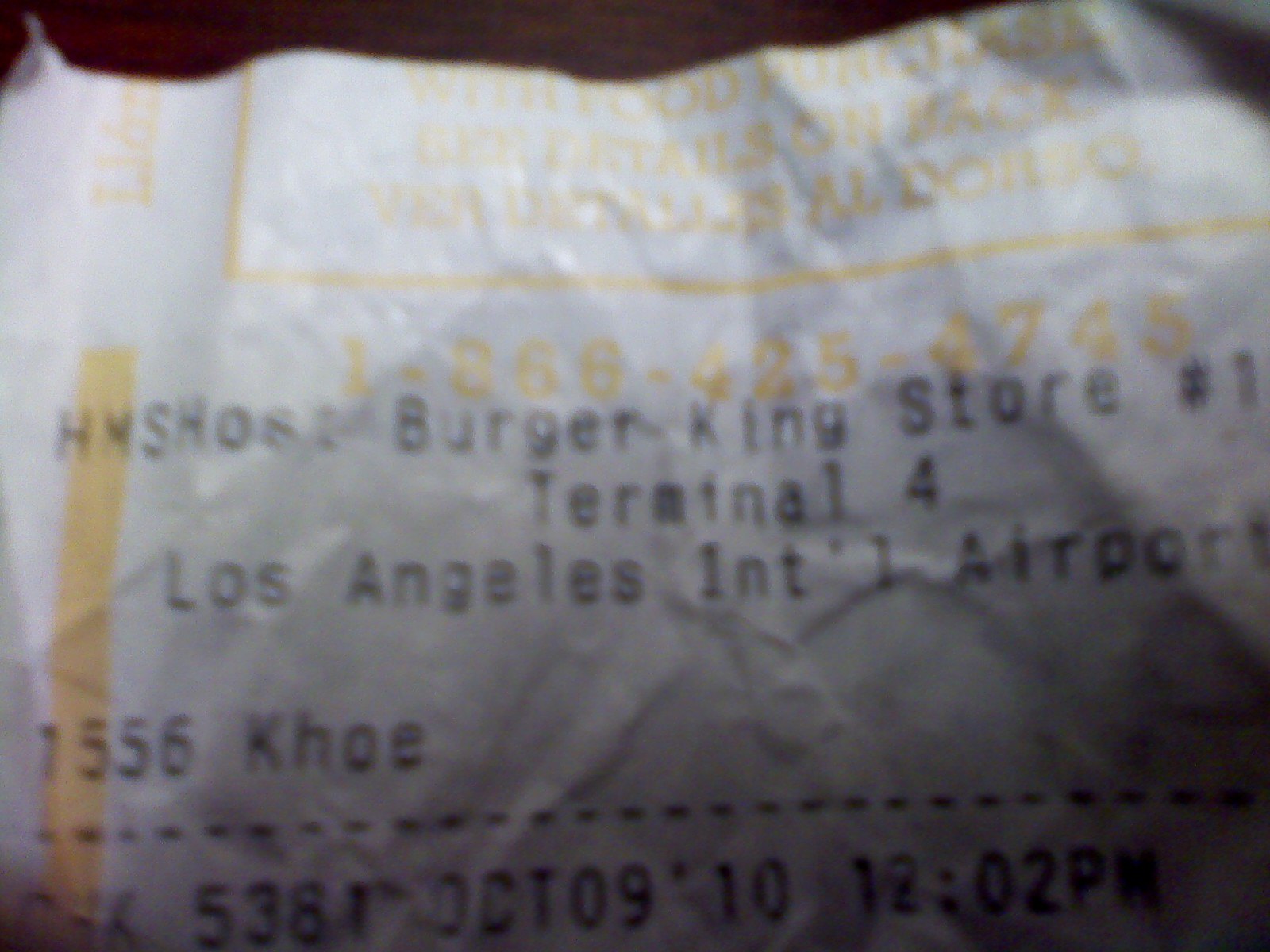This close-up photo captures a crumpled and then re-flattened receipt from a Burger King store, taken under dim lighting conditions. The image is somewhat blurry, obscuring finer details. At the top of the white receipt, printed in black, it reads "Burger King" followed by "Store Number: 1". Below this, "Terminal 4, Los Angeles International Airport" is clearly stated. Further down, the number "1556" appears next to the initials "COE". A dashed line separates this section from additional details below, which include "5381", the date "October 09, 2010", the time "12:02 PM", and a concluding line, presumably related to the transaction specifics.